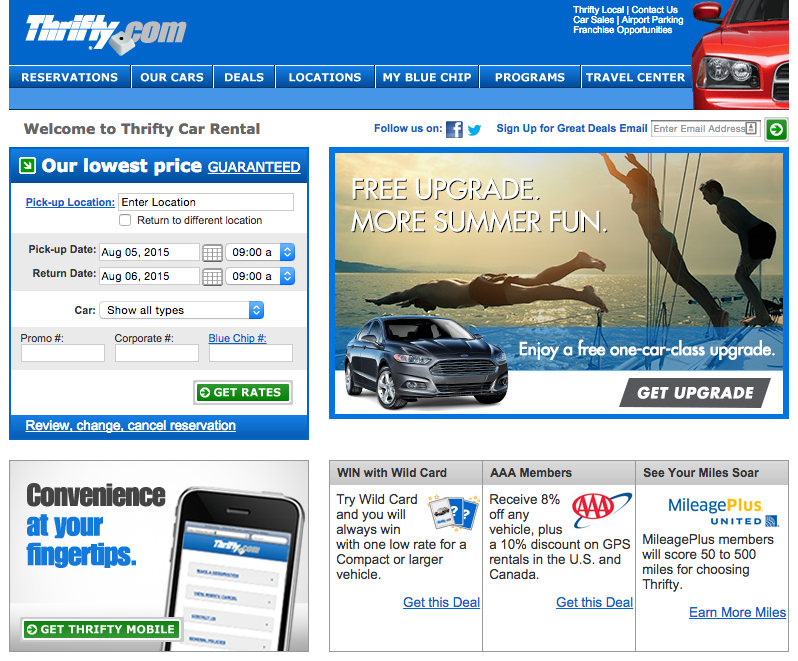This image is a screenshot of Thrifty's car rental website in landscape mode.

At the top left corner, the URL thrifty.com is displayed. The top right corner features navigation options: "Local," "Thrifty Local," "Contact Us," "Car Sales," "Airport Parking," and "Franchise Opportunities." Below is a secondary navigation bar with links to "Reservations," "Our Cars," "Deals," "Locations," "My Blue Chip," "Programs," and "Travel Center."

The webpage is divided into two main columns. On the left, there's a welcome message: "Welcome to Thrifty Car Rental." Below it are options and forms, including "Our Lowest Price Guaranteed," and fields for "Pickup Location," to enter a location, and an unchecked option to return to a different location. Pickup and return dates are both set for August 5th, 2015, and August 6th, 2015, respectively, at 9 a.m. There is an option to "Show All Types" of cars, and empty fields to enter a promo number, corporate number, or Blue Chip number. A prominent green button labeled "Get Rates" is available for guests.

The bottom left corner highlights the convenience of mobile use with the phrase "Convenience at Your Fingertips, Get Thrifty Mobile." The upper right corner encourages following Thrifty on Facebook and signing up for email deals.

Additional promotional content includes a section titled "Free Upgrade, More Summer Fun," inviting users to enjoy a free one-car-class upgrade with a gray button labeled "Get Upgrade." The bottom right corner presents various deals, including "Win with Wildcard," "AAA Members, See Your Miles Soar," with multiple "Get This Deal" buttons and an "Earn More Miles" incentive.